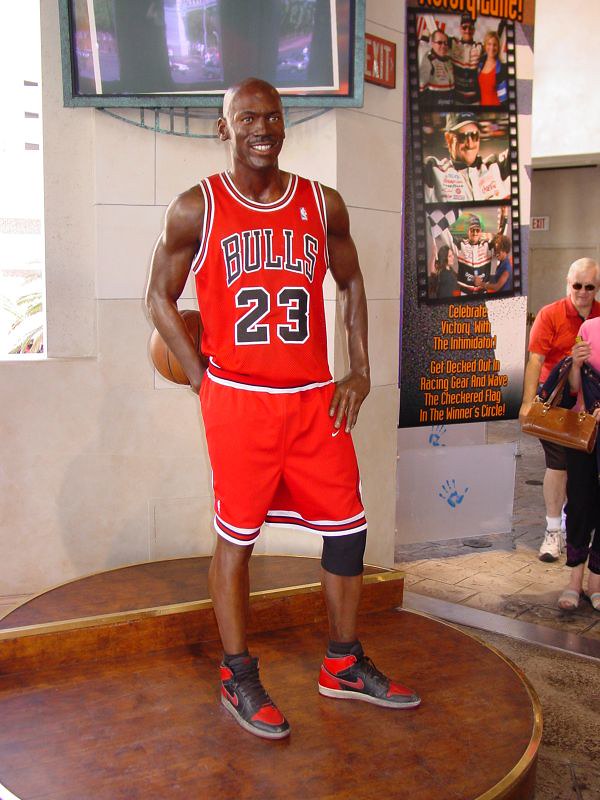In this detailed indoor photographic setting, a remarkably lifelike wax statue of Michael Jordan takes center stage, exhibited in a museum. Jordan is captured wearing his iconic red Chicago Bulls jersey with the number 23 and "Bulls" emblazoned in black on the front. The uniform includes matching red shorts, a black knee wrap reminiscent of his later career, and black and red Jordans. The statue, depicting a bald Jordan with a slight mustache, holds a basketball behind his back with his right hand while his left hand rests on his hip, standing on a circular wooden plinth adorned with gold trim.

Above the statue, a flat-screen monitor shows a reflection possibly depicting a baseball and some outdoor buildings. The background features a white cinder block wall with an exit sign displaying "EXIT" in red and white, and another exit sign in the background. To the right of the statue, there is a promotional poster filled with images of Dale Earnhardt, titled "Celebrate Victory with the Intimidator," followed by engaging call-to-action texts like "Get Decked Out in Racing Gear," and "Wave the Checkered Flag in the Winner’s Circle," along with painted handprints at the bottom of the banner.

The museum scene captures two women: one in her 40s wearing an orange shirt and black pants along with sneakers, and only the partial presence of another woman’s hand gripping a brown handbag and wearing sandals. They appear to be walking towards the camera, adding a dynamic and human element to the detailed exhibit display.